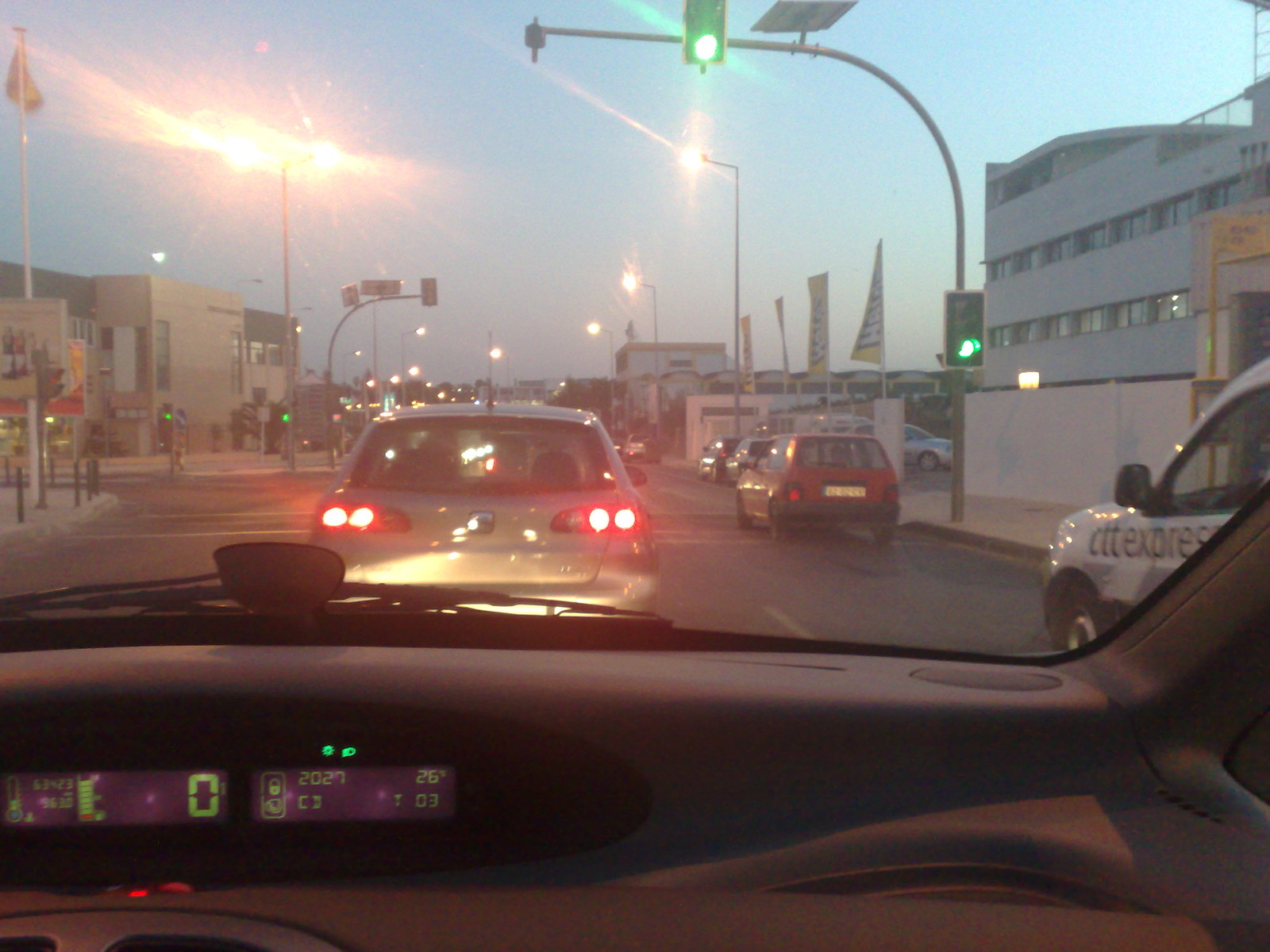This image is taken from the front seat of a car, showing the detailed dashboard and the view through the windshield. The dashboard, prominently featured at the bottom of the image, is gray with two screens. The right screen displays a number 0, a temperature thermometer, some green bars, and green text, while the left screen shows a lock icon and a number 27, accompanied by various other readings, including 26 and 3.

Through the windshield, the street scene is visible. Directly ahead, there are a couple of cars, one of them gray, stopped at a four-way intersection with green-lit traffic lights indicating go. To the right of the car, you can see the front end of a white vehicle with "CTT Express" written on it, and a red car further ahead.

On the right side of the street, there are several white buildings, one of which appears to be a car dealership, identifiable by the flags atop its pillars. To the left, additional buildings can be seen, with hints of sunset light in the background. The entire setting suggests a busy business area with multiple road lights and bustling traffic.